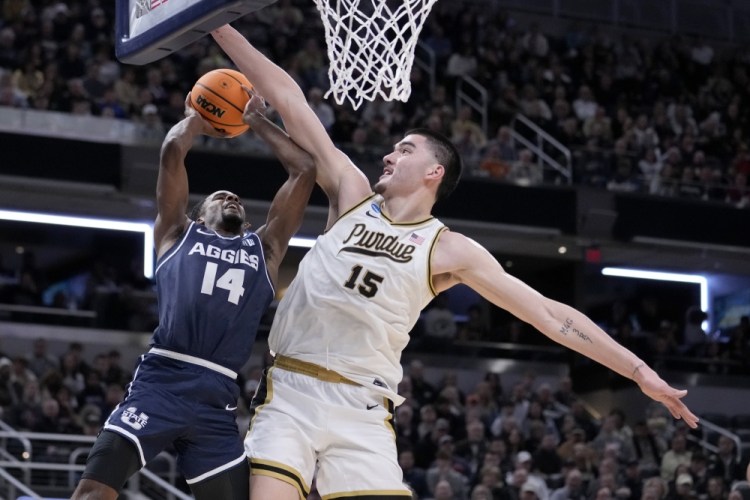This photograph captures an intense moment in a college basketball game between Purdue University and another university identifiable by their "Aggies" uniforms. In the foreground, player number 15 from Purdue, a white male with a tattoo on his left arm, is wearing a white jersey with black lettering and gold accents as well as matching shorts with green at the bottom. He is leaping towards the net with his hands stretched out wide, attempting to block his opponent. The opposing player, a black male in a blue uniform with "Aggies" in white text and number 14 beneath it, is mid-air, aiming to shoot the basketball into the hoop. The background of the image reveals a crowd of spectators seated in the stands, eagerly watching the action unfold.